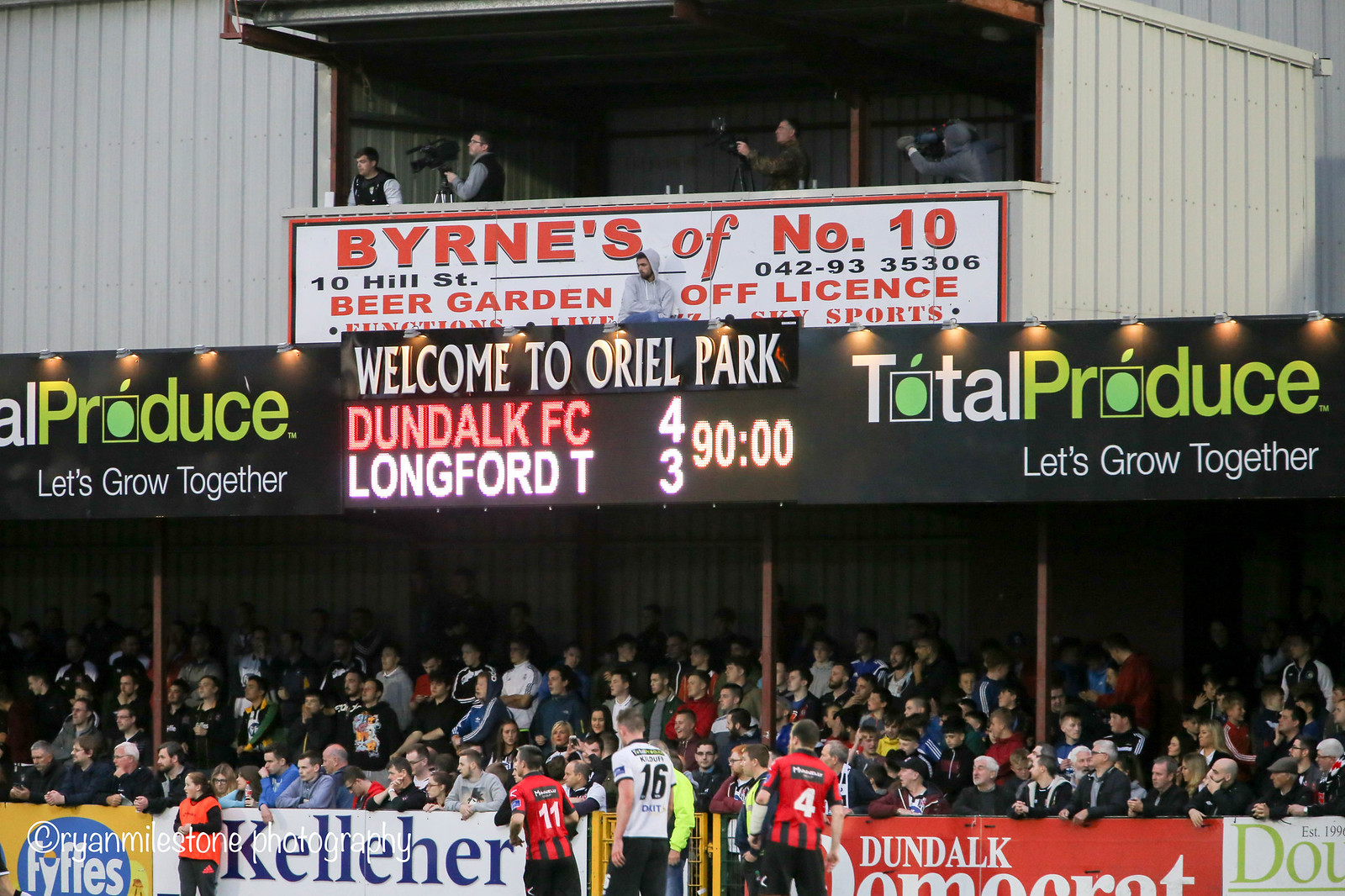The image captures the vibrant atmosphere of a soccer match at Oriole Park. The stadium's seating area is packed with spectators, showcasing two distinct levels of engagement. The lower section features rows of bleachers filled with fans, while the upper section is a balcony or press box with individuals recording the event with cameras.

Above the crowd, a white building with open awnings houses the press box. Prominent advertising signage displays "Burns of Number 10, 10 Hill Street, 042-9335306 Beer Garden, Off License. Functions, Live Show, Sky Sports." Below this is a large black scoreboard reading, "Welcome to Oriole Park. Dundalk FC 4, Longford T3," highlighting a close match with 90 minutes on the clock.

The contrasting team kits, red and black for one team and white and blue for the other, are visible although the focus is more on the stadium's lively atmosphere rather than the pitch. Additional advertisements including "Total Produce, Let's Grow Together" are seen around the seating, emphasizing the community and commercial spirit of the event.